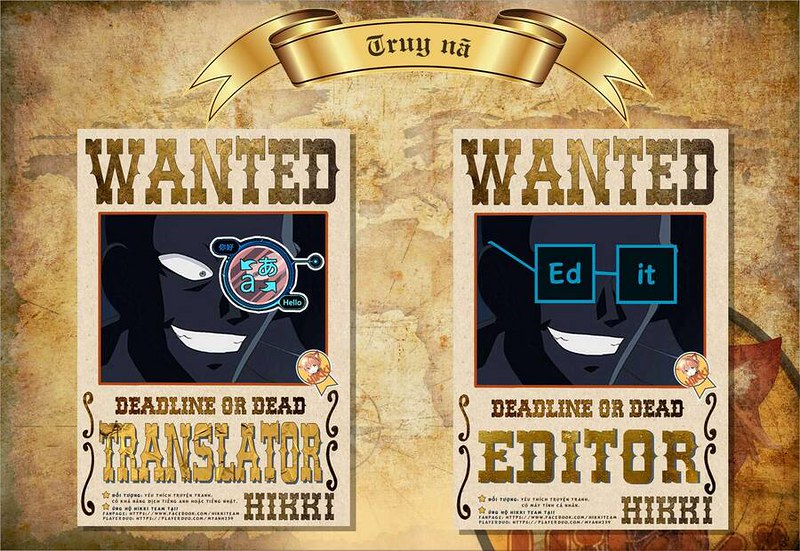The image is set against the background of old map paper, with the detailed features of the map being largely obscured and hard to discern. Overlaying this antiquated backdrop is a graphic depiction of a gold ribbon at the top, adorned with the bold, black text "TRUNYA." Below this, the image features two humorous wanted posters in a beige background and gold western-style font. Both posters prominently display the word "WANTED" at the top. The poster on the left details a blue-skinned character with a distinct large left eyebrow, an exceptionally white smile, and a right eye featuring a blue circle with a pink center and light blue Asian-style text accompanied by arrows. This poster reads "DEADLINE or DEAD, TRANSLATOR, HIKKI" at the bottom. The right poster showcases a character wearing blue square-framed glasses, with the text "Ed" and "it" displayed on the respective lens. It also reads "DEADLINE or DEAD, EDITOR, HIKKI" at the bottom. The map-paper background lends an antiquated, whimsical feel, complementing the playful, anime-styled characters on the wanted posters.